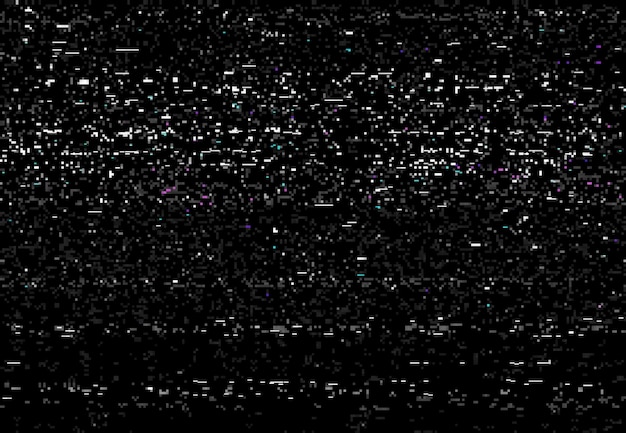This image displays a visual reminiscent of faulty, old television static, where a predominant glossy black background is sporadically covered with pixelated white, gray, and black fuzz. The upper portion of the image is heavily adorned with horizontal streaks and dots, primarily white, resembling snow. These white markings become less frequent yet still appear as faint lines and dots descending towards the bottom. Additionally, there are subtle streaks of cyan and purple interspersed within the fuzz, contributing to the overall distorted and malfunctioning electronic appearance. The image's chaotic distribution of colors and pixels vividly recalls the erratic visual noise seen on out-of-tune analog TV screens.